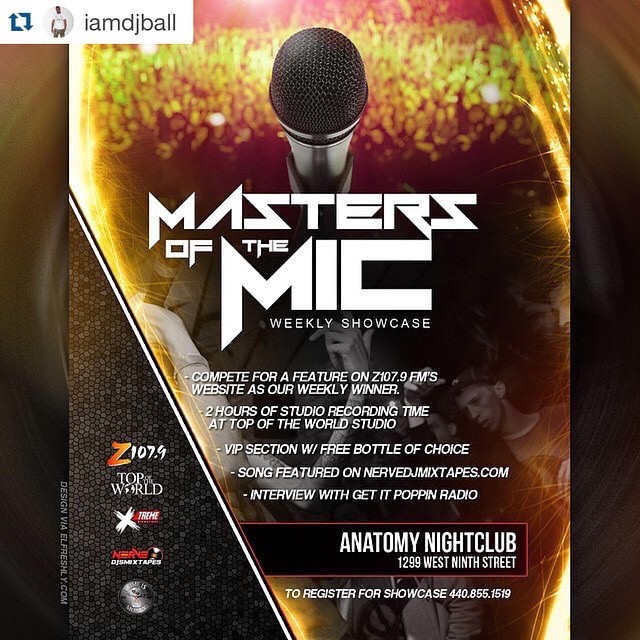The image is a vibrant, portrait-oriented promotional poster for the "Masters of the Mic Weekly Showcase" to be held at Anatomy Nightclub, located at 1299 West 9th Street. The poster combines color photography and illustration with graphic design elements, showcasing a bold and energetic aesthetic.

At the top center of the poster is a prominently featured microphone, beneath which the title "Masters of the Mic Weekly Showcase" is displayed in modern, angular, bold white lettering. The background is a dynamic gold and brown reflection of people dancing in a nightclub, seamlessly blending photographs of enthusiastic crowds from various angles.

In the body of the poster, several bullet points outline the competition's enticing rewards: a feature on Z107.9 FM's website as the weekly winner, two hours of studio recording time at Top of the World Studio, a VIP section with a free bottle of choice, the winning song featured on NERV J Mixtapes, and an interview with Get It Hot Get It Poppin' radio. These details emphasize the opportunity for participants to gain significant music industry exposure.

On the left side, the poster features the Z107.9 logo along with several other sponsor logos. In the top left corner, there is a round photo of a young man in a white shirt accompanied by green arrows forming a square, adjacent to the text, "I am DJ Ball."

At the bottom right, the poster lists the address and registration information for Anatomy Nightclub, inviting aspiring musicians to sign up and compete.

Overall, the poster effectively promotes the "Masters of the Mic Weekly Showcase" with a blend of vivid imagery and clear, enticing details to attract participants and audience members alike.